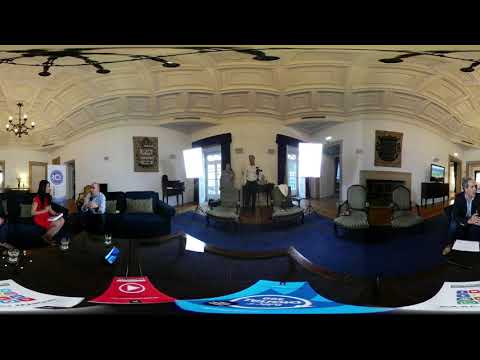This photograph, taken with a wide-angle or fisheye lens, showcases the interior of an official-looking hall or meeting room, resulting in a distorted view creating unnatural curves. The room features a coffered ceiling adorned with intricate white plaster work and fancy chandeliers hanging from above. The setting suggests an older building with a sophisticated ambiance, further emphasized by the details of the white and cream ceiling design. The floor is covered in a navy blue carpet.

In the image, multiple individuals are seen dressed in formal or business casual attire. A man in a black business suit sits on a couch on the left side, appearing to be engaged in an interview or conversation with a woman in a red dress seated across from him. In the middle of the room, there's a platform area with two gray chairs positioned in front of it, resembling a stage setup. Additionally, on the far left, another man is observed sitting with his arms resting on his knees, seemingly conversing with someone outside the frame. A fireplace can also be spotted in the background, adding to the room's formal atmosphere. The photo is bordered by a black banner at both the top and bottom, although no readable text is visible. The overall setting conveys a sense of an official or governmental environment.